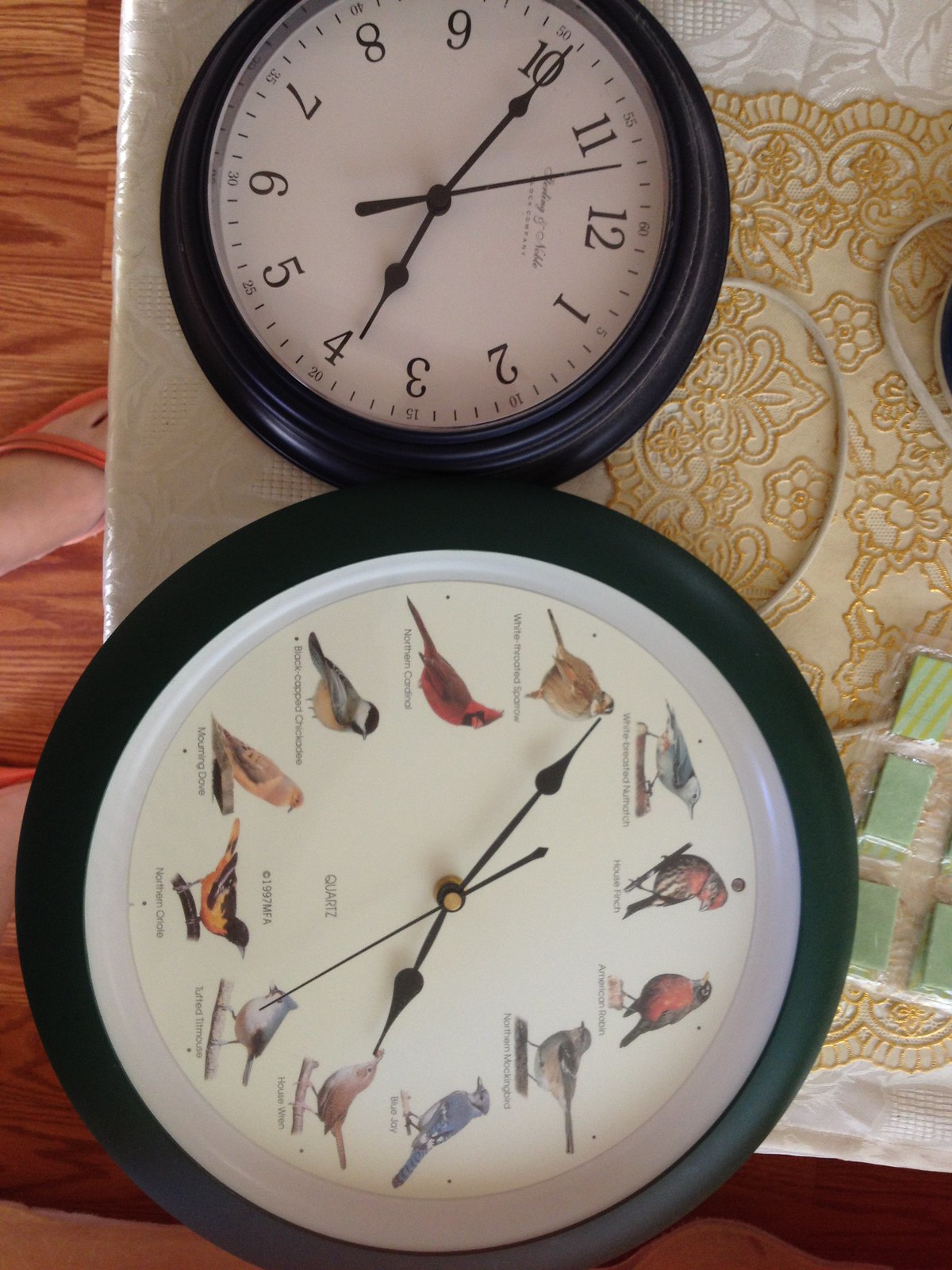This detailed photograph captures a serene scene featuring two distinctive clocks displayed on a table draped with an elegant white and gold-laced doily. Behind the clocks, a delicate white ribbon is partially visible, along with several small strips of material, one of which features white and yellow stripes.

At the top of the image, a classic round black clock stands out with its crisp white face, black numerals, and black hands. Contrasting this, at the bottom of the image, is a whimsical bird clock. This clock is also round and black with a white face but uniquely decorated with images of various bird species, each vividly colored and positioned at different hour markers. The hands of the bird clock are sleek and black, echoing the design of the first clock.

A closer inspection reveals a glimpse of the surrounding environment: a section of wood flooring, a person's foot clad in an orange flip-flop, adding a casual, human element to the otherwise still life composition.